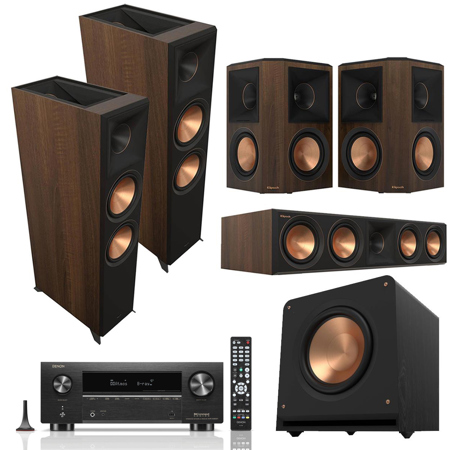The image showcases a collection of audio equipment set against a white background. The setup prominently features two tall, rectangular speakers with black fronts and wood-grain sides, housing copper-colored speaker cones likely purposed for bass frequencies. In addition, there are smaller speakers, similarly designed with copper-colored cones and probable tweeter units, suggesting they handle higher frequencies. A notable component is a larger, black box-shaped subwoofer equipped with a significant speaker, estimated to be around 10 to 12 inches in diameter, designed for deep bass sounds.

Central to this arrangement is an amplifier-receiver unit, which is gray in color and features two large control knobs, possibly for volume and tuning. Accompanying this unit is a substantial remote control with numerous buttons. Another distinctive speaker is square-shaped with a bronze-gold center, while a rectangular, flatter speaker showcases a configuration of four drivers, including two smaller ones, likely for mid-range and high frequencies, surrounding a central tweeter.

This ensemble of audio equipment, with its retro aesthetic and varied speaker sizes and types, hints at a comprehensive surround sound setup, possibly ideal for a home theater experience.